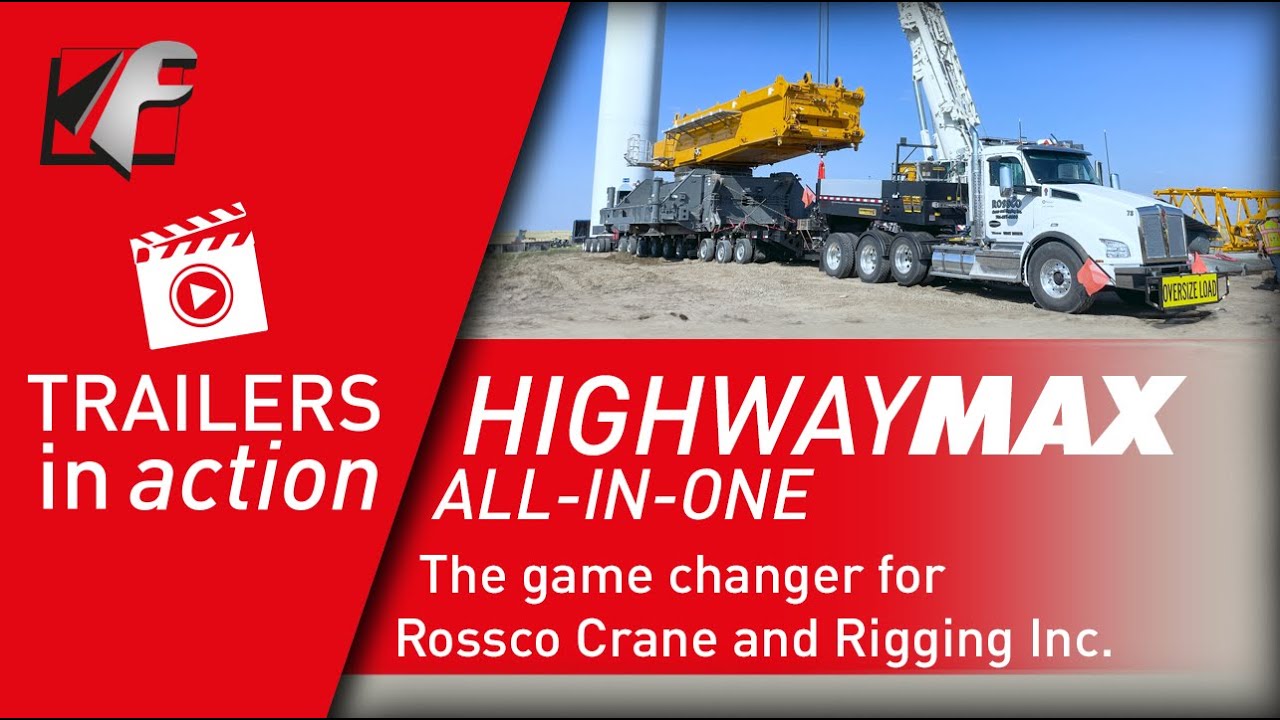The image is an advertisement dominated by vibrant colors and text. On the far left, a red background features a logo resembling a gray wrench and a red square with a black triangle beneath it. Below this, a movie-style clapboard icon with a play button and the text "Trailers in Action" appears in white. The central and right parts of the image showcase a scene under a clear blue sky with no clouds, where a white semi-truck labeled "Oversized Load" is hauling a substantial yellow crane atop a wheeled platform, reminiscent of tank tracks. In the background, there's a tall, white cylindrical silo. The ground beneath the truck is dirt, contributing to an industrial setting. Overlaid text on a red banner reads "Highway Max All-in-One: The Game Changer for Roscoe Crane and Rigging Inc" in white, emphasizing the key message of the advertisement.